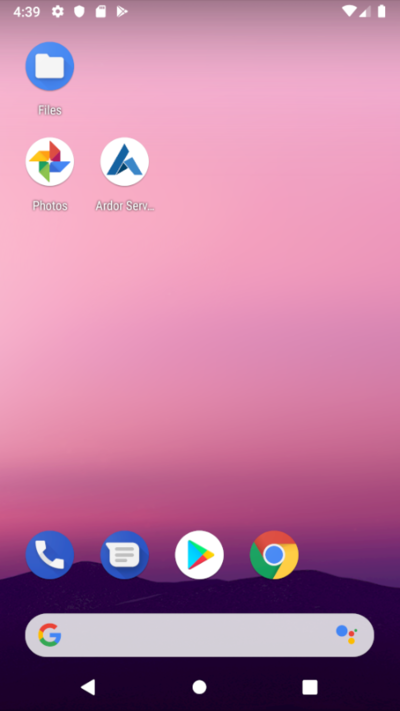This screenshot features a gradient pink background, indicative of a modern and sleek aesthetic. At the top of the screen, several icons are visible: a standard file icon, the Google Photos icon, an icon for Adobe services, and the Chrome browser icon, depicted as a small mountainside. Additionally, familiar utility icons such as a phone icon, a message icon, the Google Play Store icon, and a Google search bar appear.

The screenshot seems to be from an Android device, as suggested by the layout and icons. The current time displayed is 4:39. Also visible are icons for settings, a shield suggesting security features, a small arrow, and a battery indicator, providing information on device status. The Google logo is present along with three small dots, possibly indicating a menu or additional options.